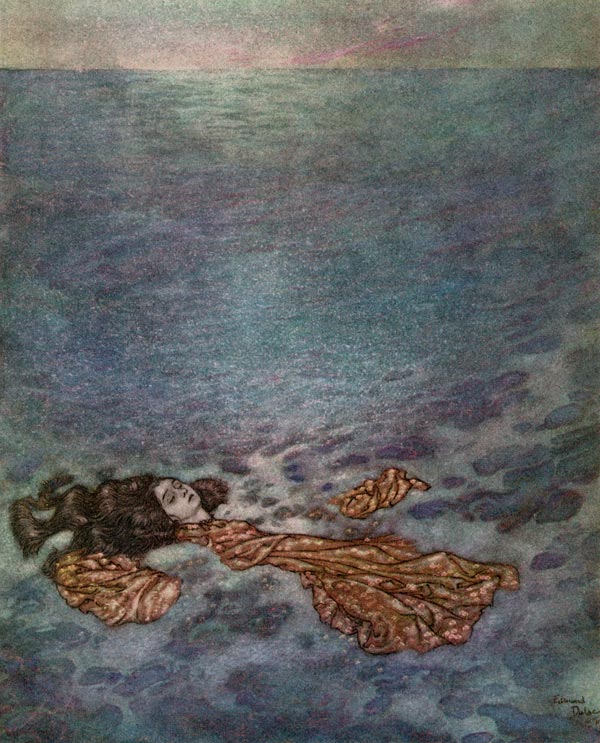The painting depicts a woman floating on her back in the ocean, surrounded by a rich palette of colors that gradually shift from the bottom to the top. At the bottom of the image, the water has a foamy, sea-green texture. The water around her body appears white, mimicking foaming waves. As you move upwards, the colors transition through various shades of blue, purple, teal, and aquamarine, culminating in a horizon line where the ocean meets the sky. The sky itself is depicted with muted, pastel hues of pink, yellow, and gray, adding a serene, almost ethereal quality to the scene.

The woman at the bottom of the painting wears a brown or red and white patterned dress which spreads out in sections around her as she floats. Her long, black or brown hair fans out behind her, and she has a white face with her eyes closed, contributing to her peaceful demeanor. The painting has a slightly cartoonish yet realistic style with a muted, blurred effect, emphasizing the dreamlike quality of the scene and the woman’s serene position in this oceanic expanse.